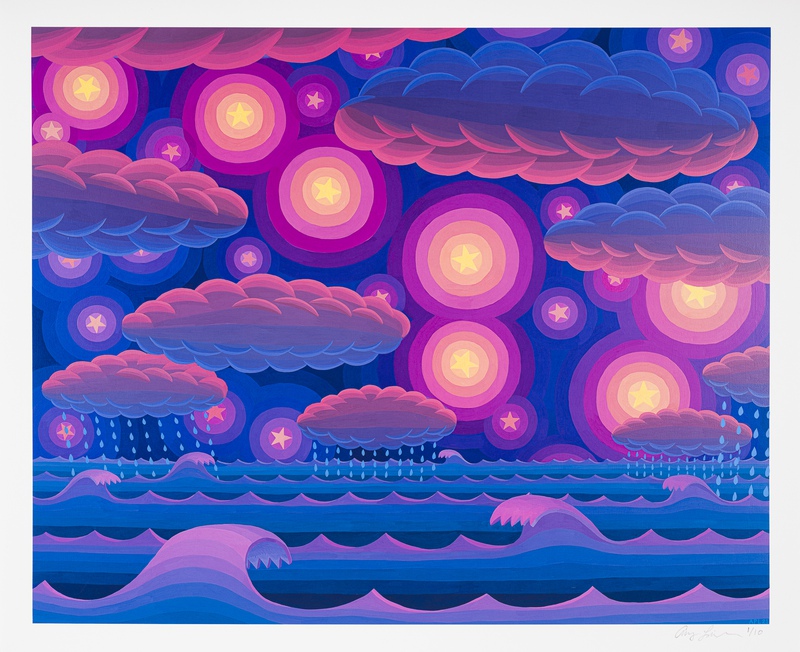This vibrant digital artwork features a vivid palette of purples, pinks, and blues. The top section showcases fluffy, two-dimensional clouds shaded in gray with blue and pink hues. Amongst the clouds, numerous circular targets are peppered throughout the image, each with concentric rings of varying colors: a purple outer ring, followed by hot pink, regular pink, light pink, peach, and finishing with a central yellow star. In total, there are at least seven of these detailed target circles. Additionally, the composition includes raindrops falling in linear patterns from some clouds, set against a vivid blue sky background. The lower portion of the image depicts geometric ocean waves in shades of blue and purple. White stars encircled by hues from yellow to orange add whimsical touches, contributing to the picture's playful, almost poster-like aesthetic.